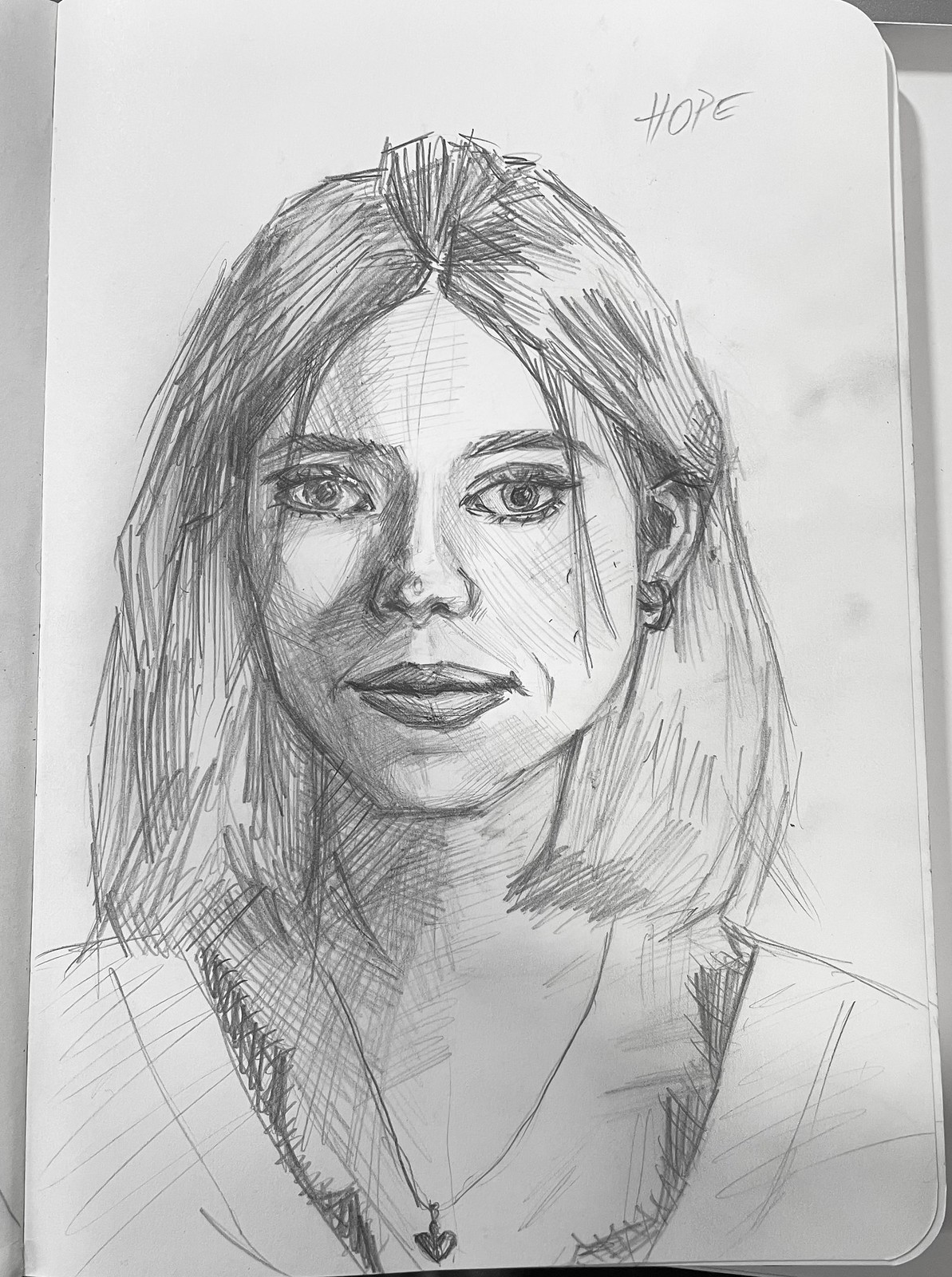This detailed pencil drawing depicts a wistful and melancholic woman portrayed from the head and shoulders. Her straight, shoulder-length hair appears thick and is neatly parted in the middle, with the left side tucked behind her ear, revealing a small hoop earring. Above her head to the right, the name "Hope" is inscribed in pencil. The woman’s face is delicately crafted, showcasing her full lips, large expressive eyes with defined eyebrows, and long eyelashes that suggest the application of eyeshadow. She has a few stray bangs draped thoughtfully across her face. She wears a lacy v-neck shirt and a thin chain necklace with a heart pendant. Her distant gaze, complemented by her slight head tilt, contributes to the overall daydreaming and somber impression conveyed by the portrait.